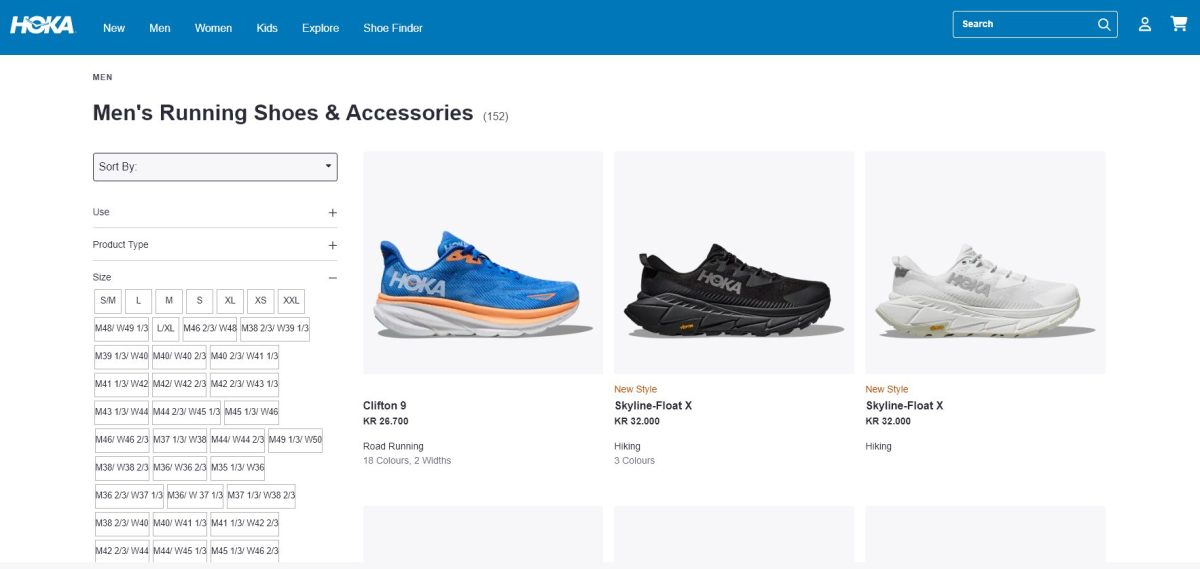This image captures a section of the Hoka website, specifically dedicated to men's running shoes and accessories. At the top, the navigation bar offers several categories: New, Men, Women, Kids, Explore, and Shoe Finder, alongside utility icons including a search bar, an account icon, and a shopping cart icon on the top right. The page prominently displays the title "Men's Running Shoes and Accessories," noting that there are 152 items available.

On the left side of the page, there is a sidebar for sorting and filtering options. Users can choose to sort the products via a dropdown menu, and further refine their search by selecting product type, usage, and size options among several listed.

Displayed on the right are product listings with detailed images and descriptions. The first product shown is the "Clifton 9," priced at KR 26.700, potentially in Krones. This shoe is designed for road running and available in 18 colors and 2 widths. The displayed image features a blue shoe with orange and white accents. Following this, the "Skyfloat X" is listed at KR 32.000, categorized as a hiking shoe, available in 3 colors. An additional image shows a variant of the Skyfloat X in white.

Overall, the image highlights the website's layout with filtering options on the left and detailed product images on the right, offering a snapshot of the available items and their specifics.